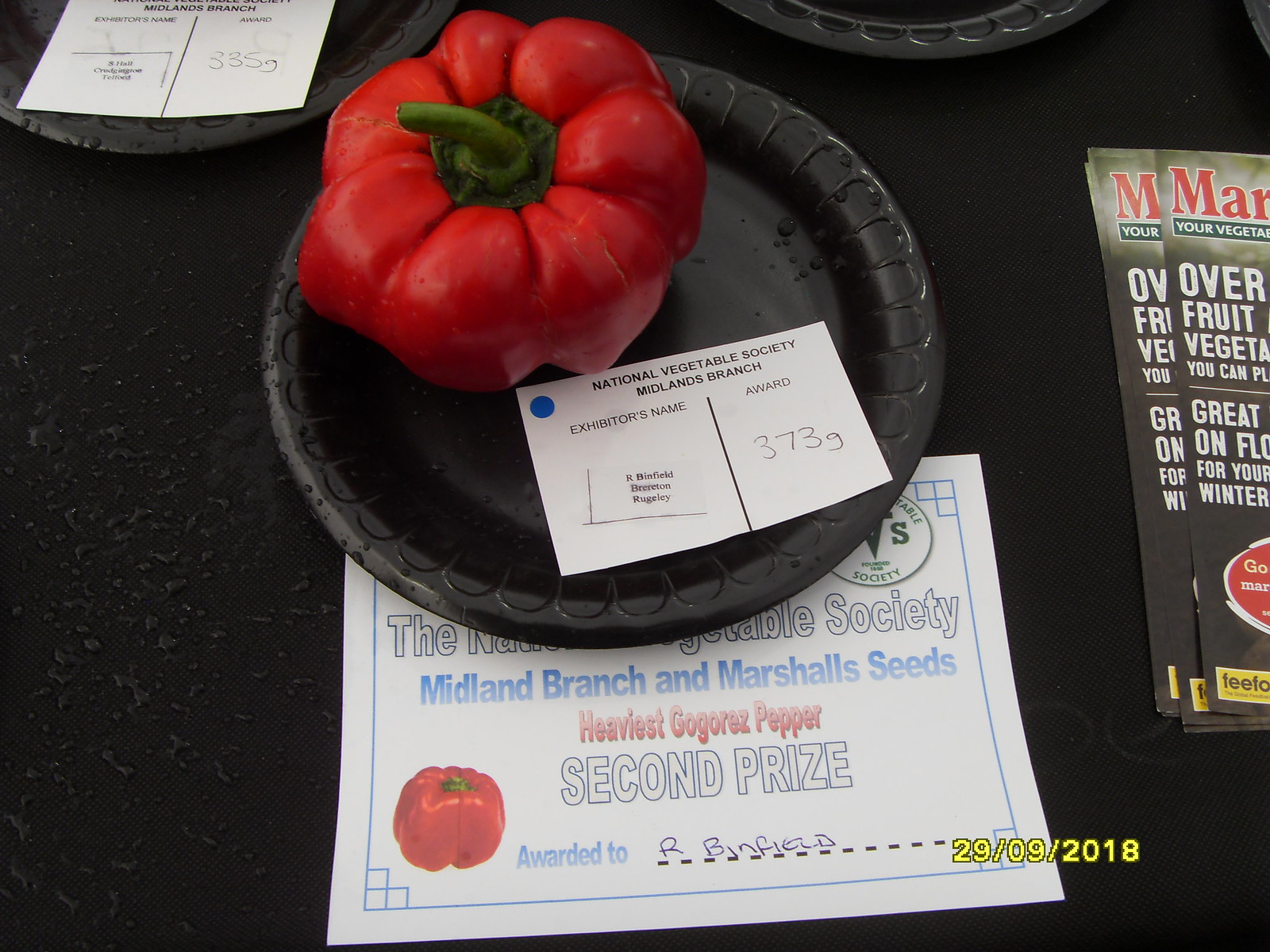The image showcases a horizontal rectangular scene from a vegetable exhibit at the fair. The focal point is a black disposable plate placed on a black table, featuring a large, vibrant red pepper with a green stem. A white card on the plate reads, "National Vegetable Society Midlands Branch," along with the exhibitor's name, R. Binford Barretton Rugley, and the weight of 373 grams. Below this plate, a white paper with blue writing states, "Midland Branch and Marshall Seeds, Heaviest Gogorez Pepper, second prize," awarded to R. Binfield. This document also includes an illustration of the pepper. To the right, partially visible seed packages or brochures add to the setting, while another plate with a tag is seen on the upper left. The detailed display highlights the pepper's achievement of winning second place in the contest.